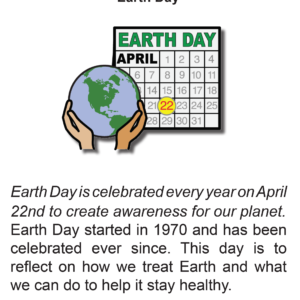In the image, we observe a detailed depiction of a globe being held by two hands, symbolizing care for the planet. The globe prominently displays North America in green, with South America partially visible but somewhat obscured at the bottom due to the positioning of the hands. Adjacent to the globe, there is a square featuring the words "EARTH DAY" in bold, green capital letters. Directly below this, another square contains "APRIL" in all caps, alongside a calendar for the month, displaying dates from the 1st to the 31st. The 22nd is highlighted with a red circle, emphasizing the importance of this date. Beneath the calendar, a caption reads: "Earth Day is celebrated every year on April 22nd to create awareness for our planet. Earth Day started in 1970, and has been celebrated ever since. This day is to reflect on how we treat Earth, and what we can do to help it stay healthy." The hands holding the globe are positioned with one on the left and one on the right, cradling the globe gently in their palms, evoking a sense of protection and responsibility.